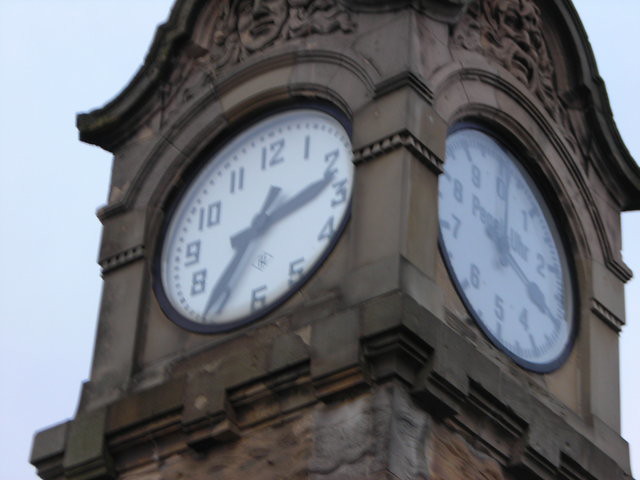This detailed photograph captures an outdoor clock tower made of stone, displaying two clock faces on its visible sides. The tower's stone surface is intricately carved, featuring arches and elaborate designs above each clock, including distinct faces sculpted in the stone — one appearing to smile slightly and the other resembling an angry man. The clock on the right has a traditional design with a white face, black hands, and standard black numbers, displaying the time as 2:35. In contrast, the clock on the left has an unconventional layout: its black numbers and white face show digits from 10, 1, 2, 3, 4, 5, 6, 7, 8, and 9, missing the usual 11 and 12. The placement of numbers is unusual, with the 3 positioned where the 4 typically would be, and the 5 where the 6 normally is. This clock also has an inscription beginning with "P-E-R," followed by "U-H-R," adding to its distinctiveness. Despite some visible indications, the exact purpose of the left clock remains ambiguous. The image does not show the entire height of the tower, limiting the view to just the section containing these ornate and unique timepieces.